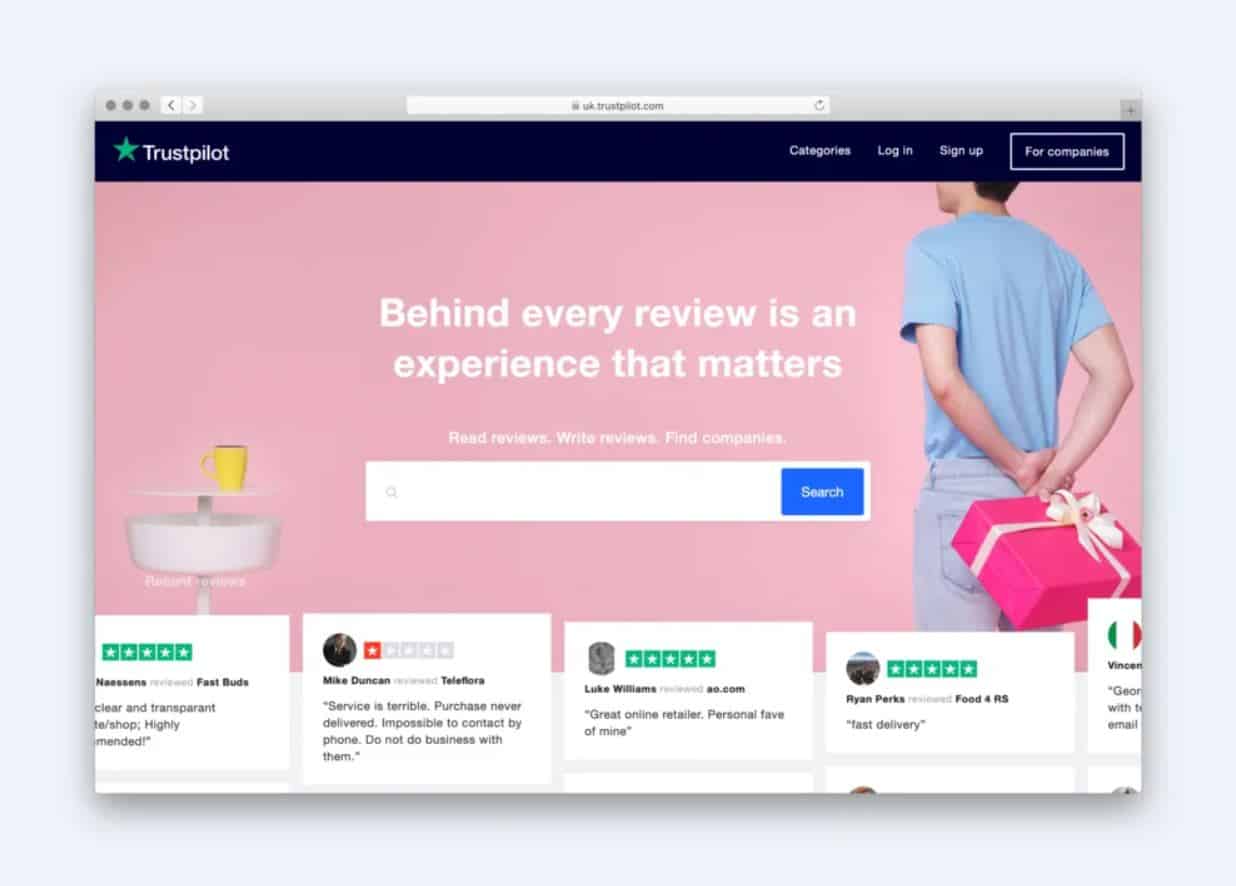The image is a meticulously cropped screenshot from a web browser, set against a plain grey backdrop that frames the screenshot itself. The browser's white address bar at the top displays the URL "uk.trustpilot.com." 

Within the homepage screenshot, a dark blue rectangle spans the top, housing the website's navigational menu and logo. The Trustpilot logo is positioned in the top left corner, featuring a green star icon alongside the text "Trustpilot" in white. Adjacent to the logo, the navigation menu offers three distinct options: "Categories," "Login," and "Sign Up." Additionally, there is a selectable rectangle option for searching companies.

The main section of the website homepage is highlighted with a pink background and a prominently large, empty search bar inviting users to search the site. 

Central to the image is a photograph of a man standing with his back to the camera, holding a pink present behind him. 

The bottom portion of the screenshot showcases a series of user reviews, complete with star ratings and brief descriptions, adding a touch of community feedback to the overall layout.